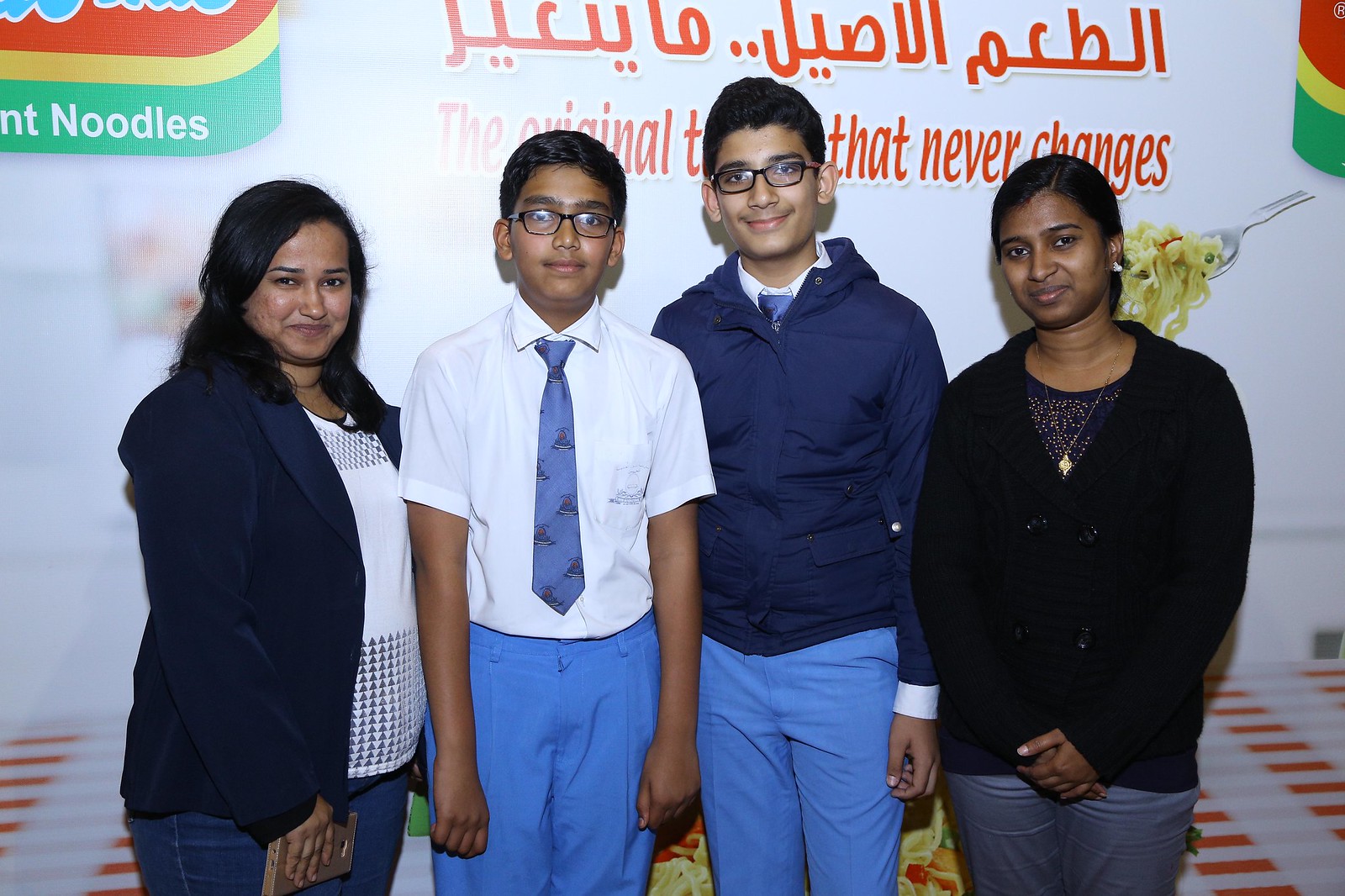This image features four Indian individuals—two females and two males—standing in front of a backdrop, which prominently displays a spoon with noodles next to text in both English and another language. The English text clearly reads "the original that never changes" with the word "noodles" also visible on the top left. The backdrop appears to advertise noodles. In the foreground, the males, who look like they are in their early teens, both wear white shirts, blue ties, and blue pants, with one of them also sporting a blue jacket. Both boys have glasses and similar hairstyles. The females bookend the group, with one older female wearing a white shirt and a blazer, and the other younger female donning a black jacket and a necklace. The attire of all individuals is notably formal.